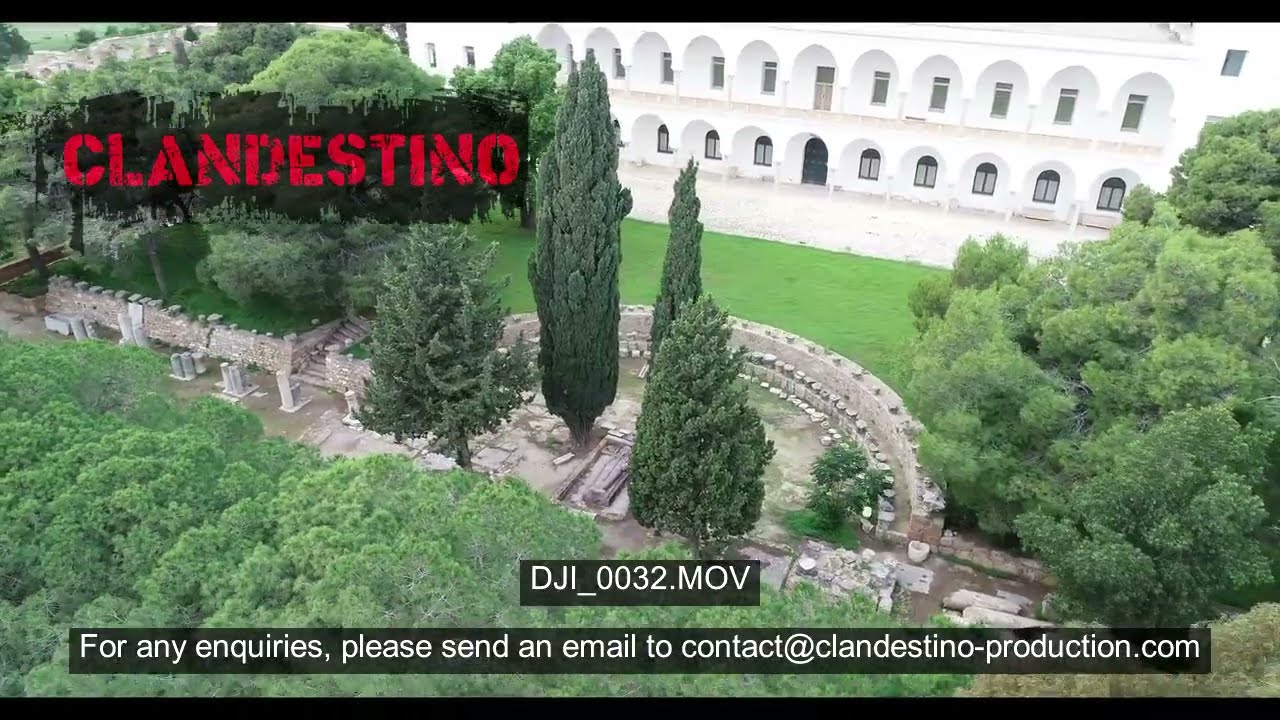A top-down aerial view captures a serene garden or park area, dominated by a large, bright-white building, possibly of North African or Middle Eastern architectural style, with its distinctive arched windows and doors. Surrounding the building is a manicured lawn and several walkways adorned with standing stone pillars and various topiary trees, creating an elegant landscaped space. The garden is further enclosed by a stone fence and features several stone monuments along its pathways. 

The image, which appears to be a screenshot from a video due to the horizontal black strips at the top and bottom, showcases the word "CLANDESTINO" in large, bold red lettering in the upper left corner. At the bottom, on a black background, white text includes a file name "DGI_0032.MOV" and provides an email address for inquiries: contact@clandestino-production.com. The scene is tranquil, with no people or vehicles in sight, leaving the focus entirely on the exquisite landscaping and architecture.